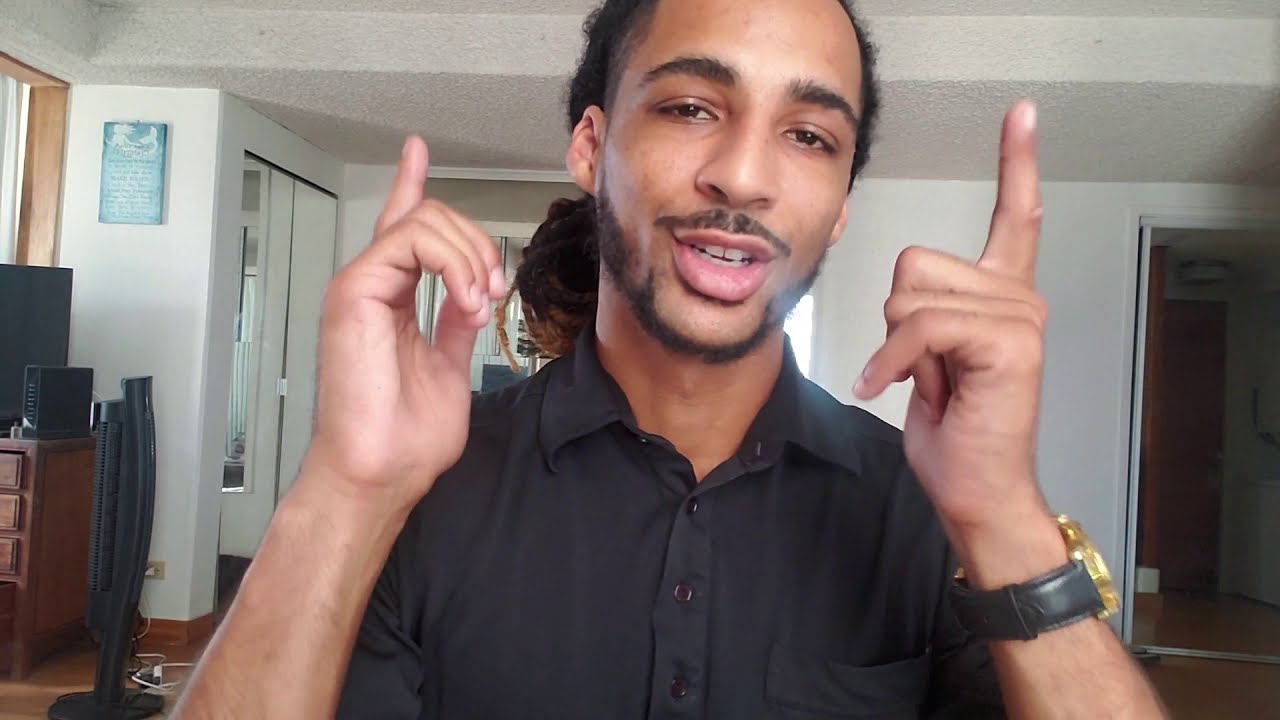The image captures an African-American man with long, braided black hair pulled back into a bun, a thin mustache, and a neatly trimmed beard. His brown skin and dark brown eyebrows frame his expressive face, where his mouth is slightly open, revealing his white teeth as he talks while looking directly at the camera. He is wearing a black button-up shirt and a watch with a gold face on his right wrist. Both his hands are raised, with his index fingers pointing straight up. In the background, we see details of a room, possibly his apartment, with white walls, a wooden door, and what seems like a dresser, a TV, and some wires on the floor. To the left, there’s a standing fan, and in the far left corner, mirrored closet doors are visible. Parts of the room also show white paint on the walls and ceiling, something that looks like an air purifier, and a sign and a window on the wall.